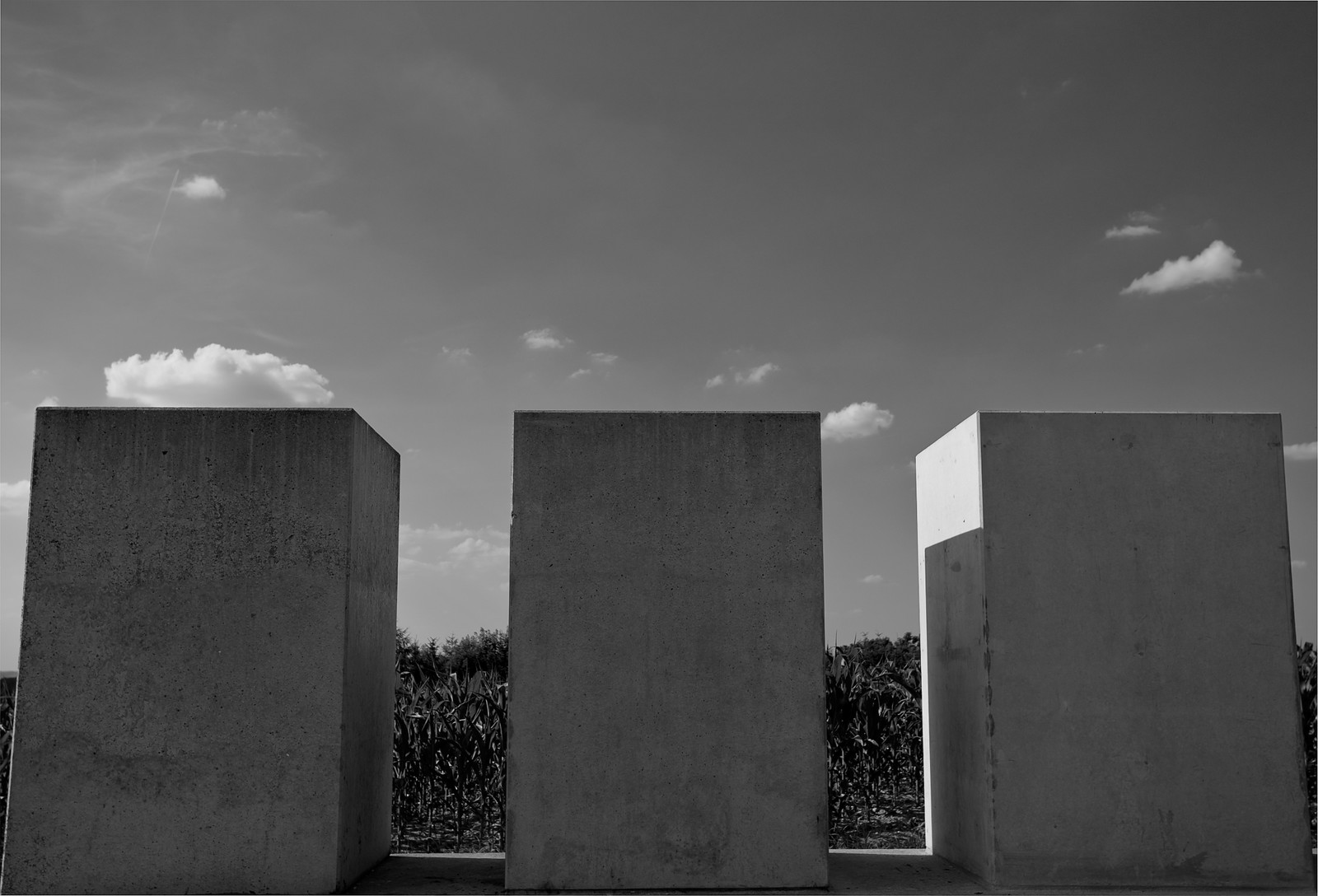In this detailed black and white photograph, we observe three rectangular cement blocks, each with identical dimensions, arranged evenly spaced apart on a concrete surface. These blocks, towering from the bottom up to about halfway through the image, cast sharp shadows, suggesting the sunlight is coming from the left. The smooth, flat-topped blocks show no readable inscriptions except for some uncertain marks on the one to the left. Behind the structures, a lush field of corn stretches, with the stalks reaching about a quarter of the height from the bottom of the picture, adding texture and depth to the scene. The sky above features a handful of clouds: a distinct, low-hanging fluffy cloud near the top left of the leftmost block, and a few scattered cumulus and cirrus clouds indicating a bright, sunny day.